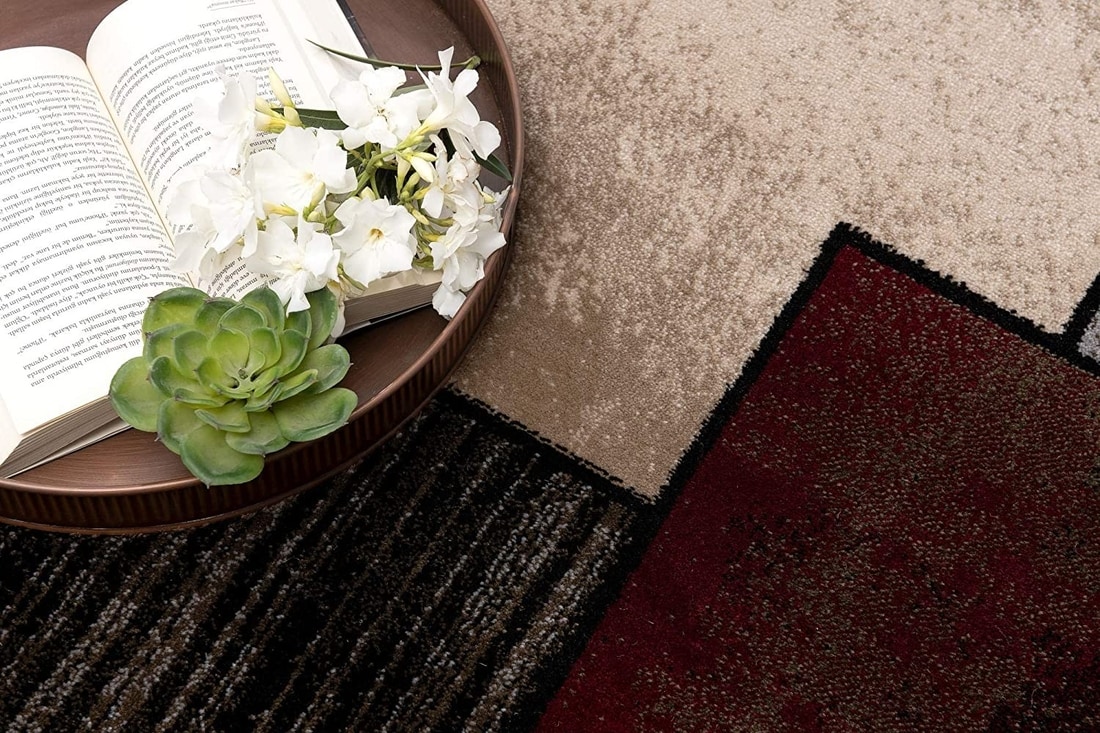This vibrant still life photograph showcases an intricate top-down view of a multi-colored carpet with distinct geometric patterns. The carpet is segmented into a tan square, a maroon square, and a multi-colored striped square, each bordered by a black outline, creating a visually cohesive yet varied design. Set against this patterned backdrop in the top-left corner is a brown wooden tray. Within the tray, a thick open book, filled with black text on white pages, lies invitingly. Draped over the right side of the book is a makeshift bouquet of several white flowers, roughly two and a half to three inches in diameter, with vivid green stems. Adjacent to these is a succulent, possibly a jade plant, adding a touch of green to the composition. The entire scene is further complemented by a bronze-colored metal plate, adding an artistic and contemporary element to the arrangement.